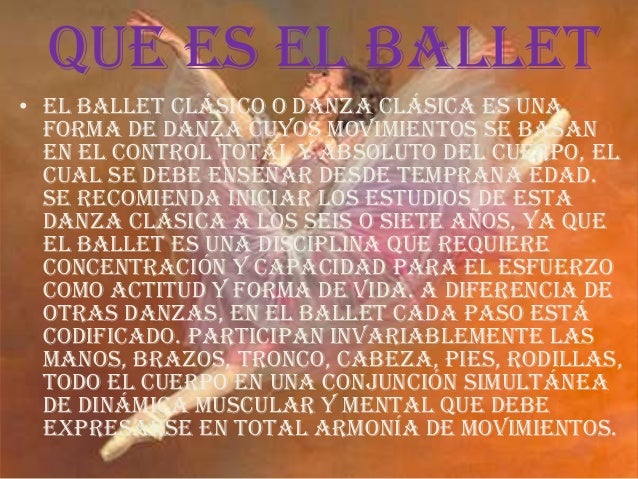The image appears to be an advertisement or poster for a ballet performance, possibly in a foreign language. The background is a gradient of orange and brown, providing a warm and inviting backdrop. At the top, the title stands out in purple, capital letters spelling "QUE EL BALLET." Overlaying this vivid background is an artful depiction of a ballerina mid-air with fully extended arms and legs, attired in white leggings and a beige dress. She has brown hair, and her poise is both graceful and powerful, embodying the spirit of ballet. The ballerina appears to be captured in a dynamic leap, her form meticulous and expressive. Beneath the title, smaller white text provides additional context, likely detailing the classical nature of the ballet and the disciplines involved, though the specifics are in a language not readily translatable. The overall effect of the poster is both artistic and informative, highlighting the elegance and dedication inherent in the art of ballet.